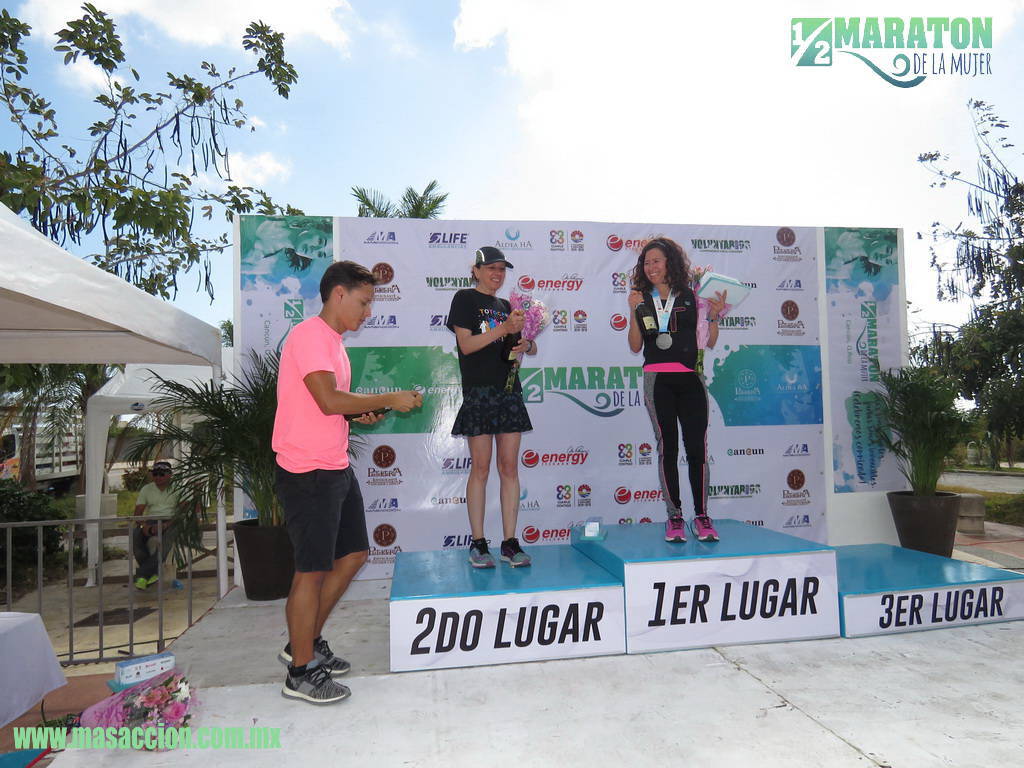In this vibrant, outdoor photograph taken on a bright, sunny day, an award ceremony is depicted for a half-marathon event labeled "1.5 Marathon De La Mujer" in the upper right-hand corner. Three women stand on a tiered podium against a backdrop of sponsor banners, with "Energy" being the most legible sponsor. The podium steps are white with black lettering on the sides, topped with blue surfaces. The woman on the tallest box marked "1ER Lugar" holds a bouquet of flowers, a bottle of champagne, and wears a large medal around her neck, signifying her first-place finish. 

Beside her on the "2DO Lugar" podium, the second-place winner also holds a bouquet of flowers. The smallest podium, labeled "3ER Lugar," stands empty. A young man with light brown skin, dressed in a short-sleeved pink or salmon-colored shirt and black shorts, is walking towards the podiums on the left, likely holding the third bouquet of flowers. The scene includes a tree to the left, a small building canopy under which a man sits, and a bright blue sky with scattered white clouds above. The setting, marked by www.masaccion.com.mx in the lower left corner, conveys a festive yet formal atmosphere typical of such events.